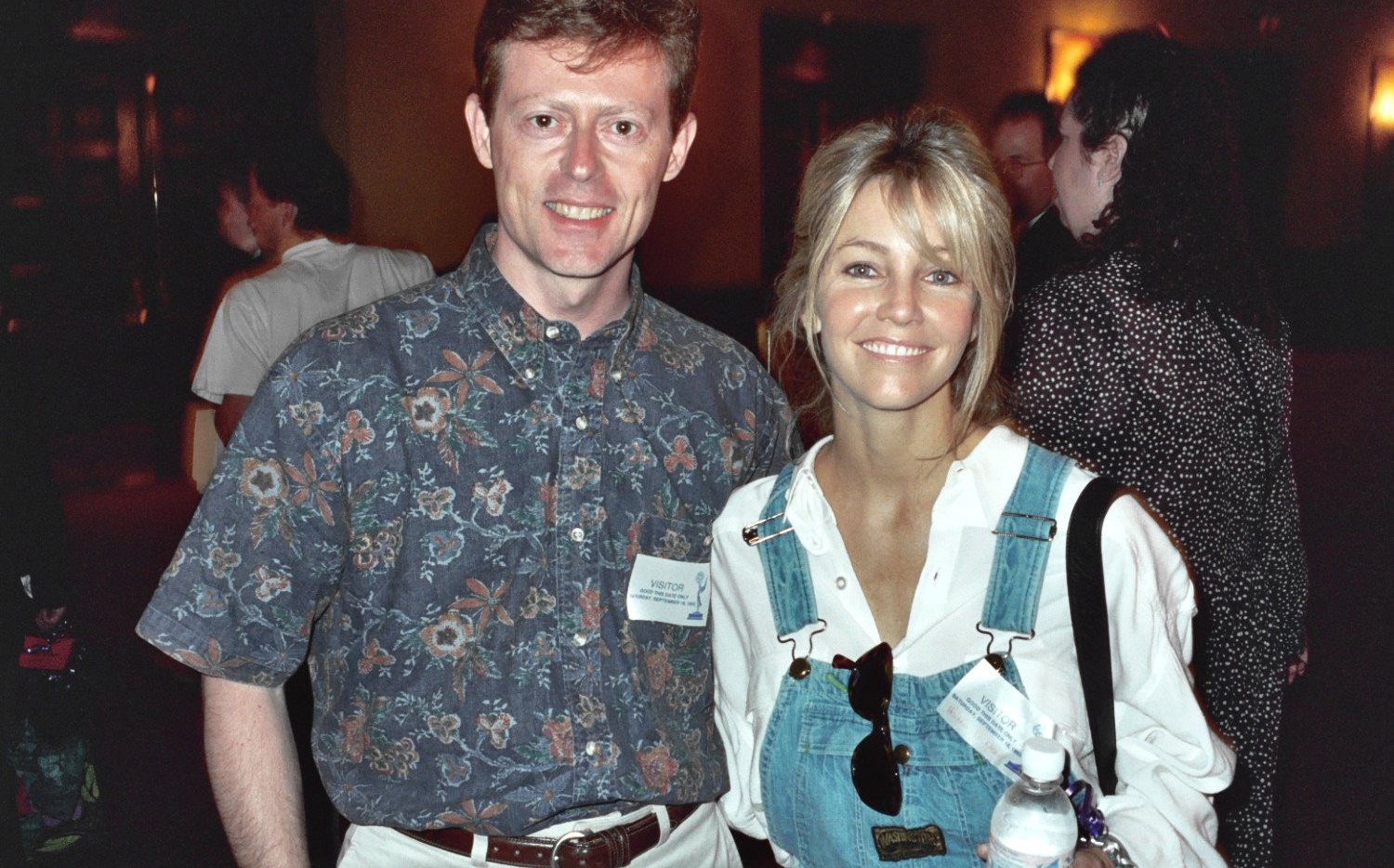In this photograph, a man and a woman are standing next to each other, both smiling warmly for the picture. The man on the left has dark blonde hair and a thin, pale face, giving him a skinny appearance. He is dressed in a short-sleeved, faded blue shirt adorned with flower designs and a white tag, paired with khaki pants and a brown belt. The woman beside him, who exudes a healthy glow akin to a model or actress, has long blonde hair with bangs swept to the side and pulled back. She is wearing a white, ruffled-looking shirt under blue denim overalls. Her outfit is accessorized with black sunglasses hooked onto the overalls and a black strap holding a white water bottle. Her makeup highlights her peachy cheeks and bright, white smile. The setting appears to be indoors, possibly a room with dark brownish tones, where the blurred backs of several other people create a sense of a busy, yet cozy atmosphere, suggesting a banquet or a similar gathering.